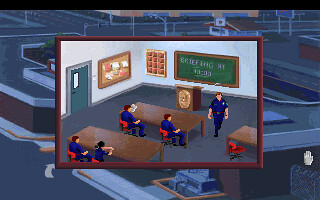The image is a complex artwork featuring two layers. The background is a city scene, possibly from a video game or cartoon, displayed as a small, square photograph with a black border across the top, as if it were a screenshot. This cityscape includes gray streets with white line markings for curbs and sidewalks, a chain-link fence in the bottom right corner, and a right-pointing arrow on the road. Structurally, there are darker buildings with white trims.

Overlayed in the center of this city background is a smaller square image with a brown, wood-tone border, depicting a classroom-like room where several figures, likely police officers, are engaged. This room has gray floors, long wooden tables, and red chairs. Four figures in blue police uniforms are seated, and one appears to be walking toward the back. The room also features a small podium, apparently with a police seal, a green chalkboard marked "briefing," and wooden cubby holes akin to office mail slots. Additionally, there's a cork board and a gray door with a small glass window near the doorknob, suggesting an institutional setting. In the bottom right corner of the entire artwork, overlapping both images, there's a small white hand symbol, emphasizing the interactive nature of the piece.